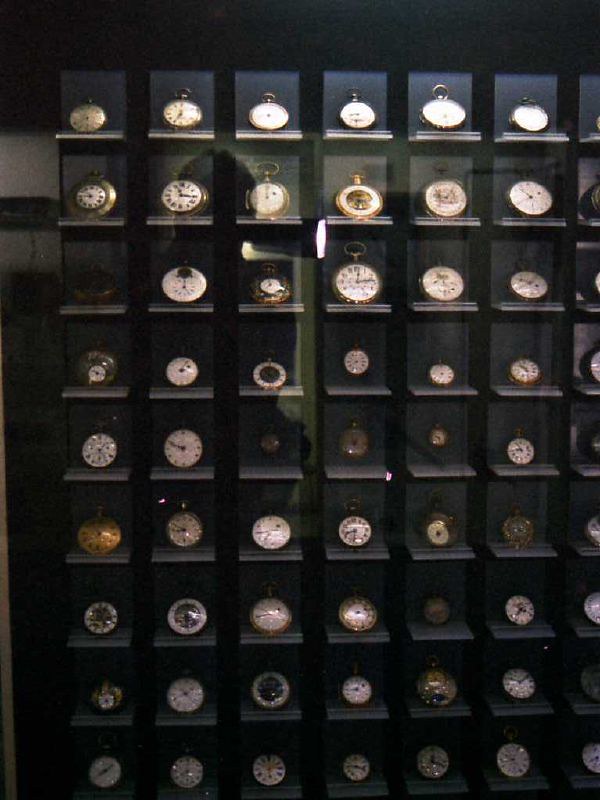The image captures a detailed display case filled with various antique pocket watches, likely situated in a museum or specialized store. The black display case, which has a glass front reflecting light, spans almost the entire frame, although we only see a portion of it. It is organized into a grid with each compartment housing a single watch, totaling nine rows down and seven columns across in the visible section. Each pocket watch, varying in sizes, predominantly features a white clock face. However, some watches boast gold or black faces. Most watches are open-faced, showcasing intricate dials and winding mechanisms at the top, while a few appear to be all metal or closed. The glass front also reflects ambient details, including a lamp, a door, part of a green wall, and the silhouette of the person taking the photograph. These reflections add depth and context to the carefully curated collection on display.